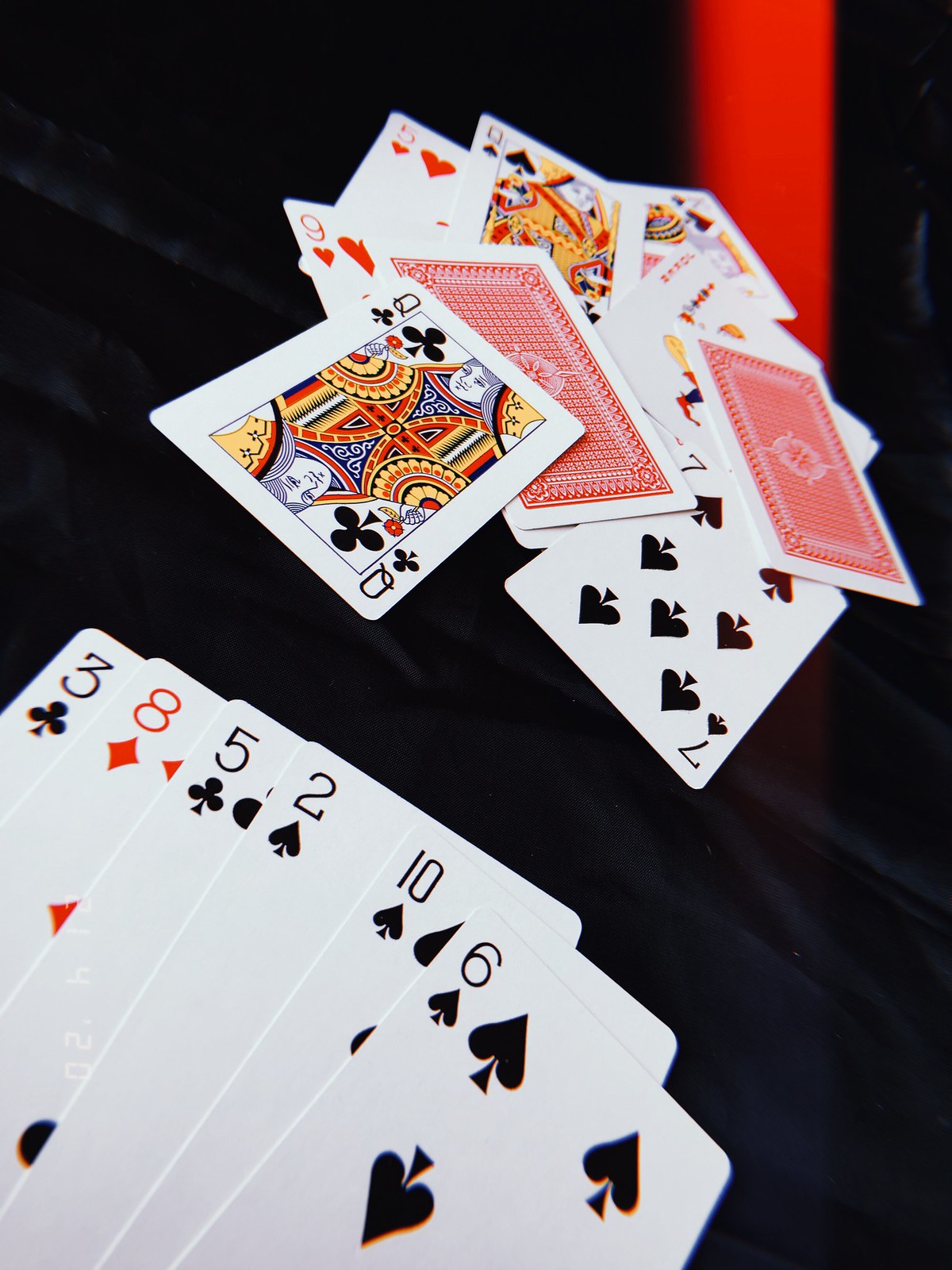The image features two sets of playing cards spread out on a black surface that resembles a comforter. The comforter, which is a dark bluish color with some wrinkles, enters from the bottom left of the image and stretches across to the right. Above the comforter, the surface is uniformly black, except for a reddish-orange streak about an inch wide that comes down from the top right, passing behind the comforter and the cards.

Starting from the bottom left corner of the image, the first set of cards is angled downward to the right. The visible cards in this set are as follows: a 3 of Clubs, then an 8 of Diamonds, followed by a 5 of Clubs. Overlaying these cards are a 2 of Spades, a 10 of Spades, and a 6 of Spades spreading towards the center top of the image. Most of these cards are face up, with two of them face down showing a red back with a white border.

The second set of cards begins with a queen of Clubs in the lower center moving upward and to the right, beneath which is a face-down card with similar red-back and white border design. Just above and slightly to the left of the queen of Clubs, a 9 of Hearts is partially visible, followed by a 5 of Hearts towards the top of the page. A queen of Spades covers half of the 5 of Hearts, and a king of Spades is barely peeking out from under the queen of Spades towards the top right. Overlapping the king of Spades are two jokers positioned side by side, with one nearly completely covering the other. Below these jokers and slightly to the right, another card with a red back and white border is partially visible. Finally, in the bottom right of this grouping, a 7 of Spades is partially overlapped by the red-backed cards.

Overall, the arrangement forms a layered, intricate spread of playing cards against a contrasting backdrop, enriched by the visual interruption of the reddish-orange streak.